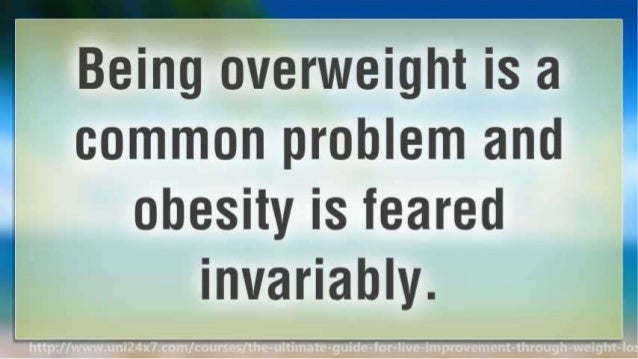The image depicts a rectangular sign with a prominent message: "Being overweight is a common problem and obesity is feared invariably." The text is in large, dark gray or dark olive green font, filling the entire space from top to bottom. The text is set against a light gray or mint green background rectangle. Surrounding this central rectangle is a larger frame featuring a scenic background with gradients of blue and white, suggesting an ocean or sky view. Additionally, there's a touch of green at the top, possibly representing tree branches. At the bottom of the central rectangle, partially cut off, is a URL: "http://www.uni24x7.com/courses/the-ultimate-guide-for-life-improvement-through-weight-loss", though the last 's' in 'loss' is missing.